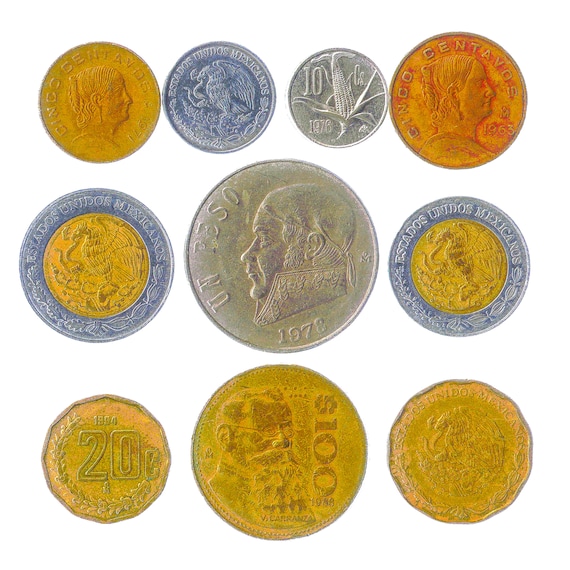In the photograph, there is a meticulously arranged collection of ten older coins against a white background, predominantly from Mexico. The coins are organized in three rows: four on the top, three in the middle, and three on the bottom. The collection features a variety of colors, including rust, purple-blue, and golden tones.

Starting from the top row, the first coin on the left is likely a Mexican peso, distinguished by its golden hue. Next to it is a silver coin showcasing an eagle grasping a snake. The third coin depicts a stalk of corn, while the fourth is a golden cinco centavos coin. In the middle row, on the left, there is another coin inscribed with "Estados Unidos Mexicanos," featuring the iconic Mexican eagle-and-snake emblem. The centerpiece of this row is the largest coin, dated circa 1978, labeled "Un Peso," with a prominent side portrait of a man in a high collar. Flanking this centerpiece are two bi-metallic coins with golden centers and blueish-silver edges, also depicting the eagle-and-snake motif.

The bottom row comprises three golden coins, identical in color to the first coin on the top row, likely suggesting a thematic consistency. The unique colors and varied designs, including heads, historical figures, and national symbols, reflect the diverse backgrounds of the currencies, making it appear like an exhibit one might see in a museum. The overall assembly of the collection emphasizes both the historical and artistic value of these coins.